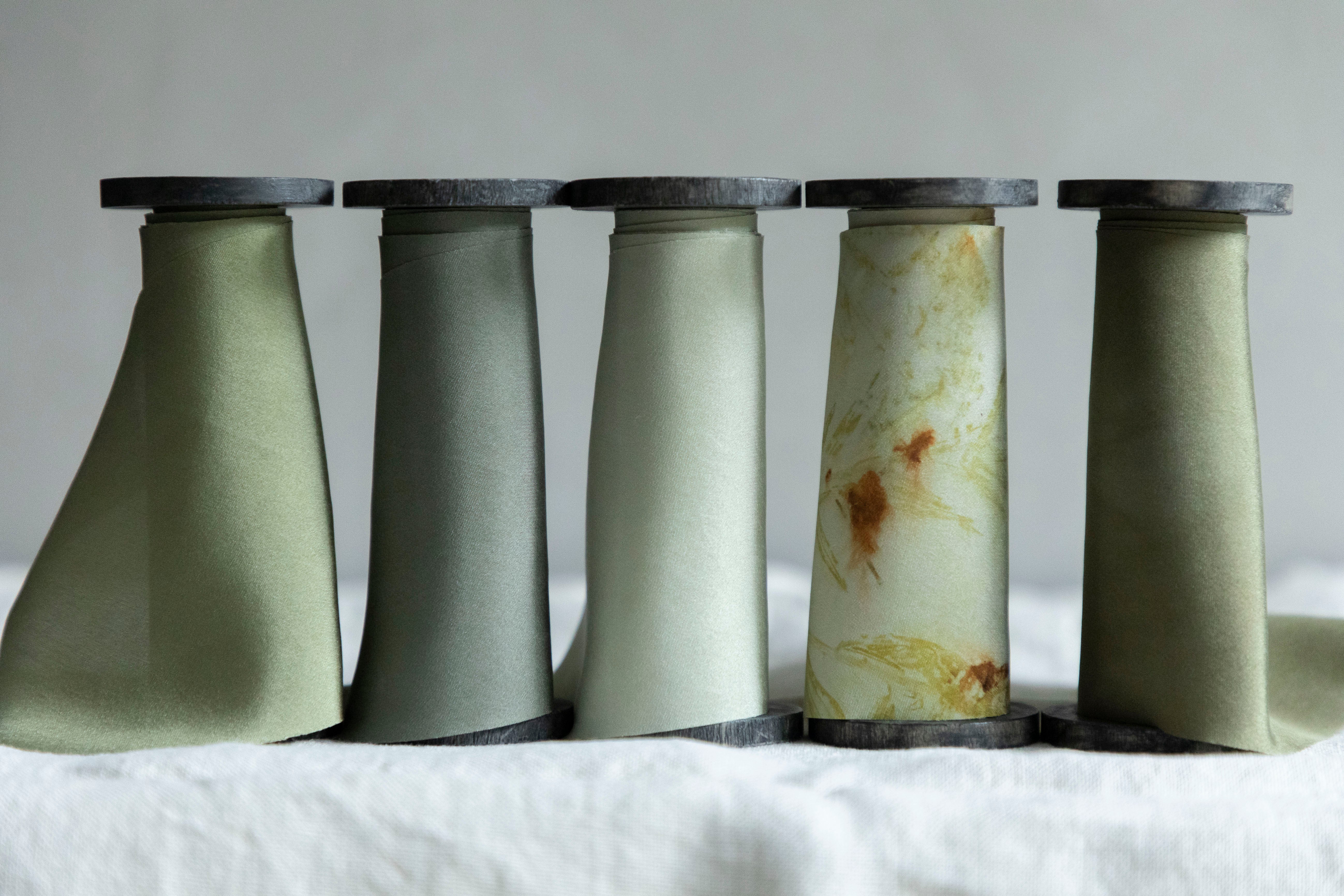The image depicts five vertically displayed spools of fabric made of a thin, silky material, likely silk, arranged on a white, cottony tablecloth against a light gray wall. The spools themselves appear to be crafted from either metal or black plastic. Starting from the left, the first spool holds a sheer, olive green fabric that delicately drapes off its side. Next to it is a spool wrapped in a dark gray material, followed by a spool featuring an ivory white fabric. The fourth spool showcases an ivory white fabric adorned with various random orange patterns, some darker than others, giving it a marbled appearance. The final spool draped in a dark green fabric completes the arrangement.